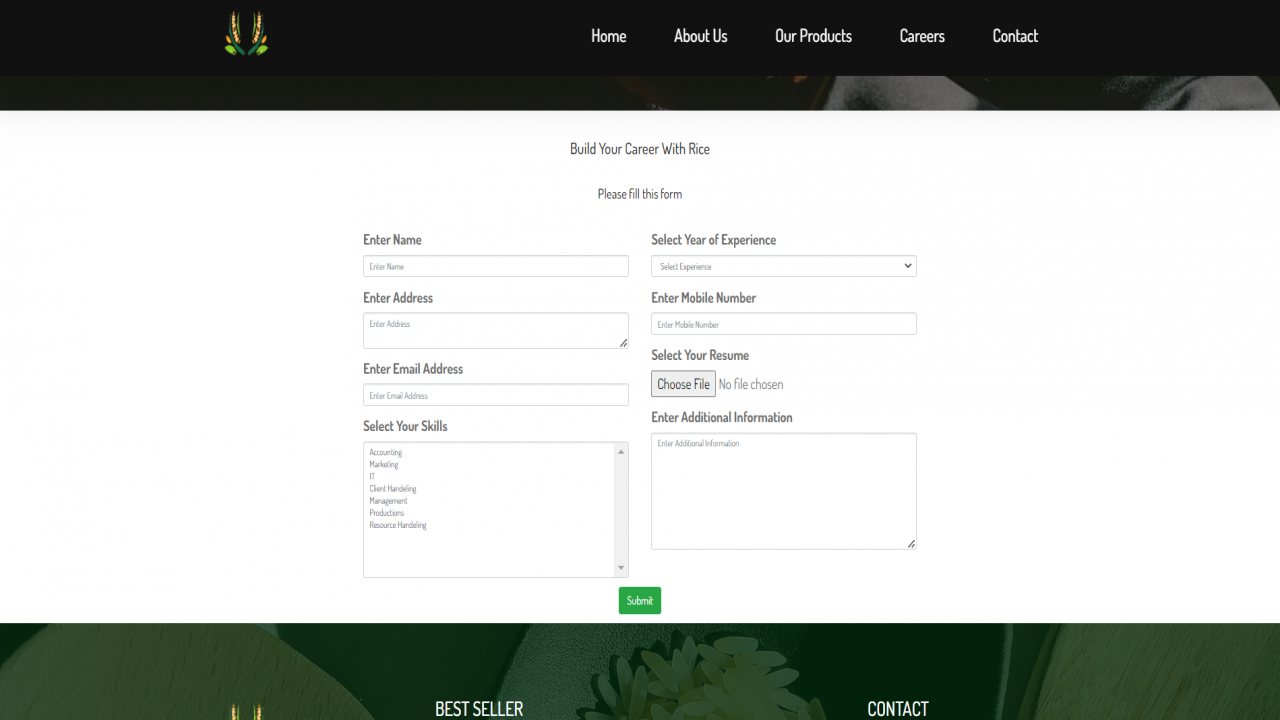The image depicts a website with a sleek design, featuring a black navigation bar at the top. The navigation bar, displaying white text, includes the following menu options: Home, About Us, Our Products, Careers, and Contact. Below the navigation bar, the webpage is primarily centered around a career application form.

The headline reads, "Build Your Career with Us." The form consists of various fields prompting the user to enter their information, including:

1. Name (Text field)
2. Address (Text field)
3. Email Address (Text field)
4. Mobile Number (Text field)

Additionally, there's a dropdown menu where users can select their skills from options like:
- Accounting
- Marketing
- IT
- Client Handling
- Management
- Product Production
- Resource Handling

To the right of these fields, another dropdown menu allows users to specify their years of experience. The form also includes a section to upload a resume, featuring a "Choose File" button indicating "No file chosen." There is an additional text field for users to enter any further information.

At the bottom of the form is a prominent green "Submit" button. Underneath, there is a light green and dark green bar with white text, stating "Best Seller" and "Contact."

Despite the detailed structure and well-organized sections of the webpage, the company's name remains unidentified, as it is not mentioned anywhere on the screen. The overall color scheme of the website includes black, white, light green, and dark green, with most informational text in black, except for the navigation bar text and the "Submit" button.